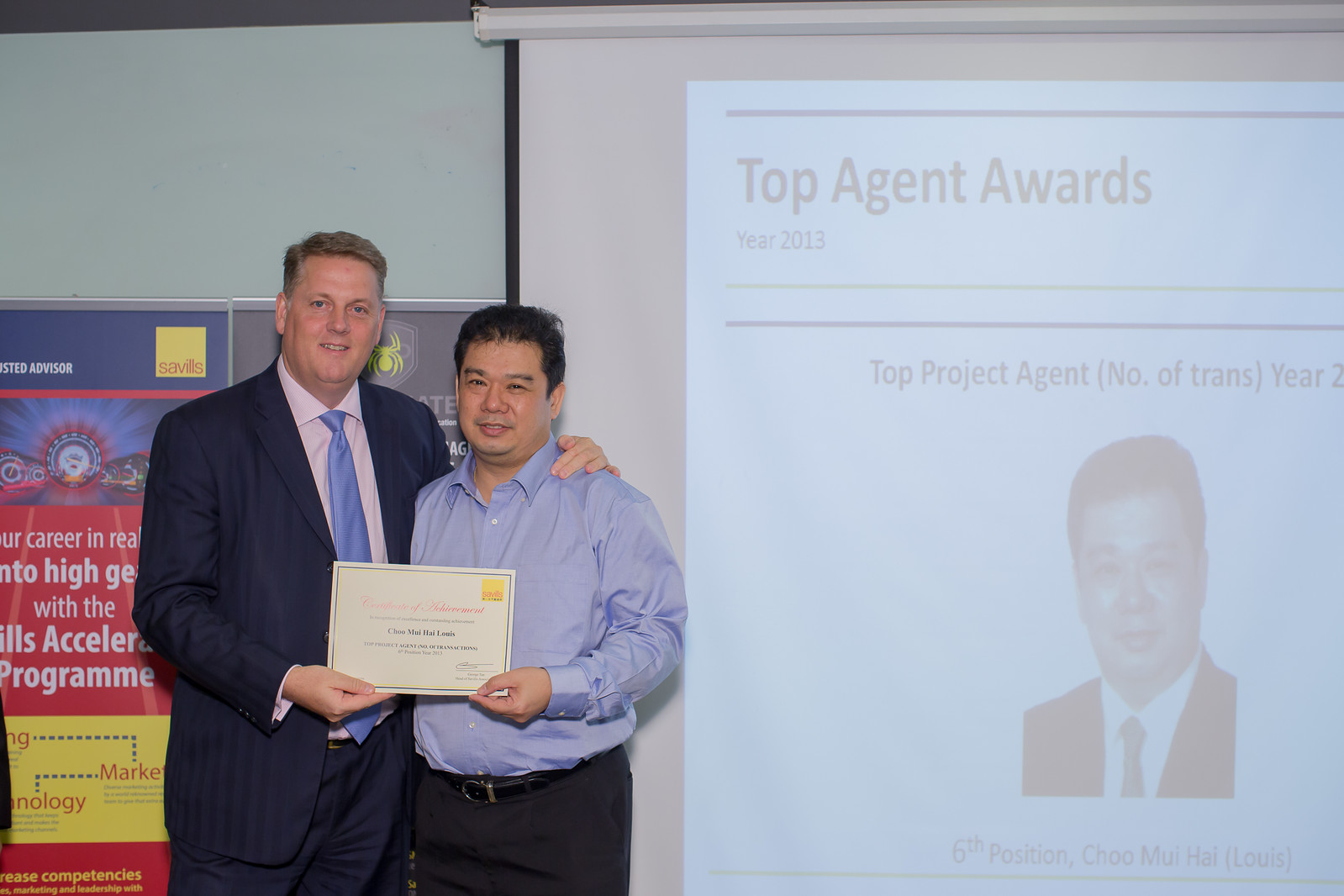In this detailed, color landscape photograph taken indoors, two men are the central focus on the left side, near the bottom of the image. The man on the left is Caucasian, taller, and has short, graying brown hair. He is dressed in a dark striped suit jacket over a pink collared shirt with a blue tie. With a double chin accentuating his open-mouth smile, he looks directly at the camera. His arm is around the shoulders of the man on his right, who has an Asian appearance, short black hair, light brown skin, and wears a blue long-sleeve button-up shirt with black trousers. Both men hold a certificate of recognition.

In the background, a partially visible sign on a light grayish-green wall appears to feature phrases like "Career in Real into High" and "Something Acceleration Program." Dominating the right side of the image is a projected screen with a light blue background displaying the text "Top Agent Awards, Year 2013." Below this headline, it reads "Top Project Agent, Number of Trans, Year 2," followed by a headshot of the Asian man. Beneath his image is the text "6th Position, Chu Mui Hai (Louis)." The scene suggests a professional awards ceremony in a business setting.